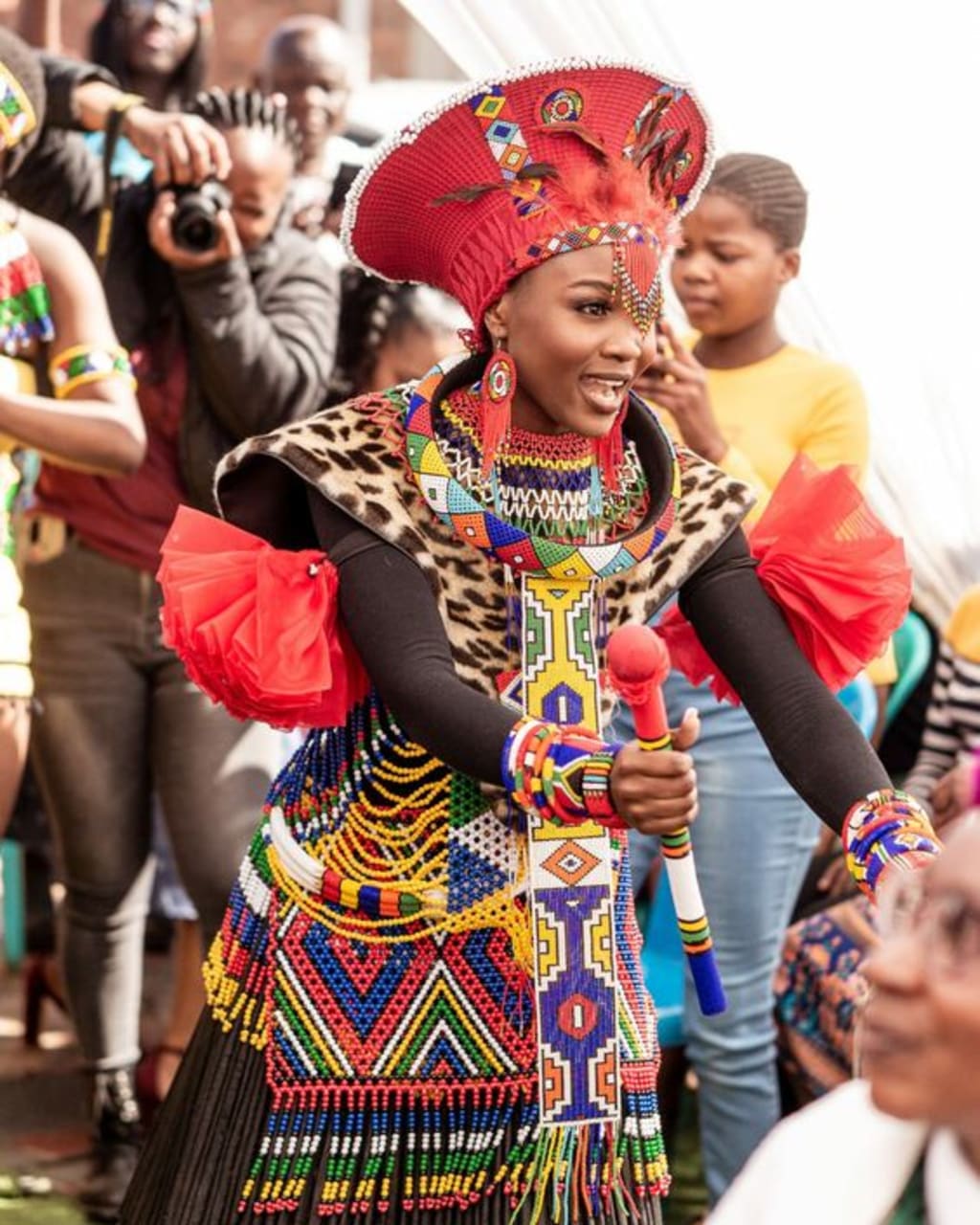In this vibrant, portrait-oriented color photograph, a young woman stands at the center, dressed in elaborate traditional Zulu wedding attire. Her striking ensemble features a vivid red hat, flared at the top and adorned with colorful triangular patterns and red feathers. Complementing her headpiece, red beads with gold tips dangle from her forehead, accompanied by long, red fringe earrings with a star pattern at the center. 

She wears a black long-sleeved top under a leopard-print vest that transitions into a beaded skirt with a fringe at the bottom, displaying a multicolored panel down the front. Her wrists are decorated with multiple colored bracelets, and in her right hand, she holds a red and white painted stick with colored bands, reminiscent of a ceremonial pole.

Capturing a moment of celebration or ritual, she faces slightly right with her mouth open, possibly chanting or singing. Surrounding her, a crowd of onlookers, dressed in casual attire, observes the scene, with one man notably taking a photograph. The lively background and detailed costume highlight the event's cultural and traditional significance, encapsulating photographic representationalism realism.